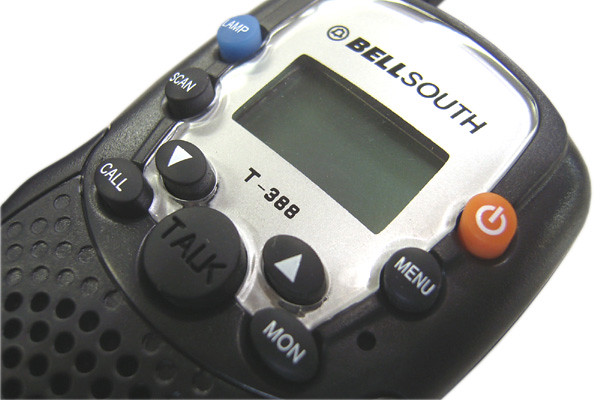The image features an older-style Bell South T-388 two-way radio, prominently displaying its brand name, "BELL south," alongside a circular bell symbol. The radio is lying flat on a white background, suggesting a photo op for advertising purposes. At the center top of the device, there's a small screen that is currently turned off. Surrounding the screen are several buttons: a blue "lamp" button to the left, and black "scan" and "menu" buttons. Below the screen, there's a larger black "talk" button flanked by a "call" button on its left and a "MON" button on its right. The buttons feature white text for easy readability. Adjacent to the screen on the right side, there's a distinctive orange power button with a white on symbol. Beneath these buttons, the speaker is visible, indicated by a pattern of small holes stamped into the sturdy, plastic surface of the radio. The entire device is colored in blue, black, white, and gray, contributing to its durable, functional appearance.